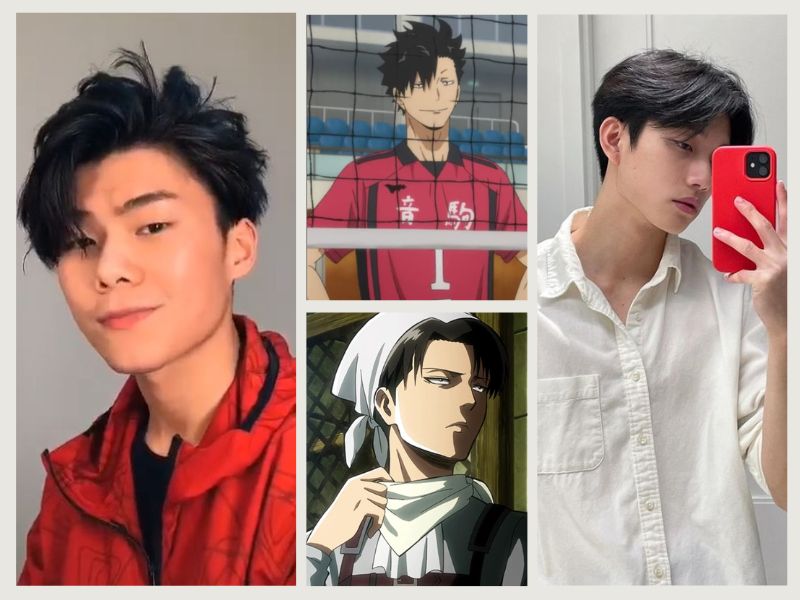This image is a composite of four distinct pictures featuring an Asian male, arranged in a rectangular layout. The far left shows a young man, approximately 17 or 18 years old, wearing a white button-down shirt with a pocket on the right side, holding up a red phone for a selfie. His head is cocked slightly to the left as he focuses on his phone. The far right features the same individual dressed in a red jacket with black trim and a black shirt underneath. His short black hair drapes over his left eye, and he gazes directly at the viewer, his lips faintly smiling. 

In the central section, two anime-style caricatures occupy the space. The upper image depicts a character resembling the real-life individual on the left, wearing a red shirt with black trim and a number, likely part of a sports jersey, visible behind a volleyball net with blue seats in the background. The lower drawing portrays another character, who appears to be the same person, dressed in a black and white outfit with a white scarf wrapped around both his neck and head, his gaze directed off to the side. These cartoon images add a creative layer to the real photographs, connecting the different representations of the individual.